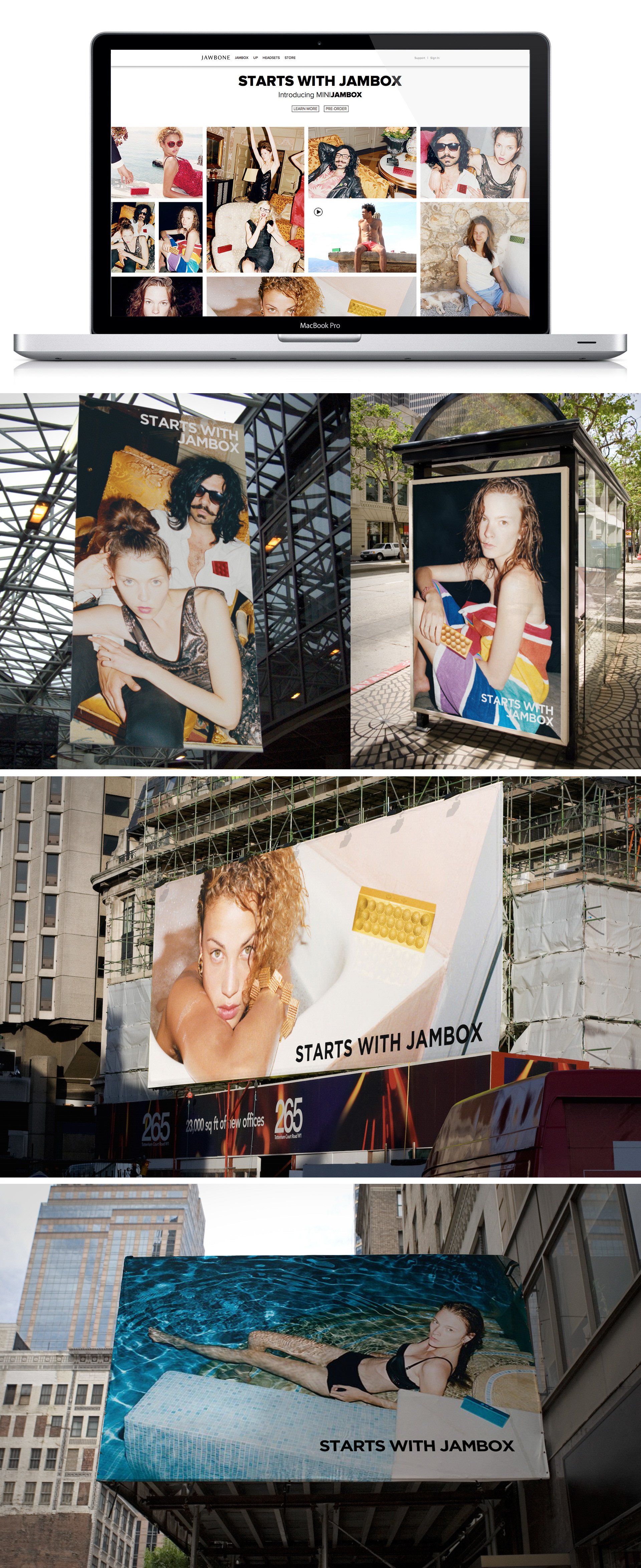The image comprises four vertically stacked frames, each showcasing different advertisements for a brand called Jambach, prominently featuring young women.

- The top frame is a photograph of an open silver laptop. The screen displays a digital collage-style advertisement reading "Starts with Jambach" in black letters at the top. The collage itself includes images of various young women.

- The second frame contains two side-by-side photographs of physical advertisements. The left side displays a banner-style ad hung from scaffolding under a glass rooftop. The ad features a woman in a black lace top standing in front of a man with long hair wearing a white suit with a red corsage. The right side shows another ad depicting a red-haired woman wrapped in a striped beach towel.

- The third frame presents a large billboard located on the facade of a department store. The billboard showcases a red-haired woman and features the phrase "Start with Jambach" in the lower right corner.

- The bottom frame captures another billboard, this time of a woman in a black bikini in a swimming pool, surrounded by blue water. The text "Starts with Jambach" is displayed beneath her.

Each frame collectively visualizes a diverse and captivating marketing campaign for Jambach, using vivid imagery and consistent branding.